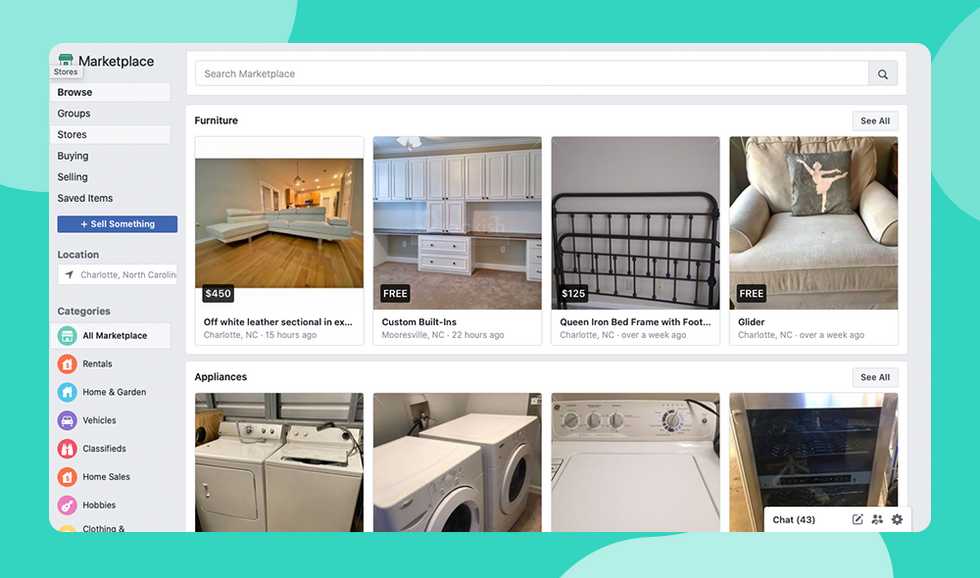This screenshot from an online marketplace showcases a platform designed for local buying and selling of various items. On the left-hand side, a navigation menu is visible, featuring categories such as Browse, Groups, Stores, Buying, Selling, Saved Items, and Sell Something, listed from top to bottom. Additionally, there is a location search bar allowing users to input their specific location for tailored search results. Below the search bar, further categories are listed, including All Marketplace, Rentals, Home and Garden, Vehicles, Classifieds, Home Sales, Hobbies, and a partially obscured Clothing category.

In the center of the image, several items for sale are displayed with detailed descriptions and prices. An off-white leather sectional in excellent condition is listed for $450, available in Charlotte, North Carolina. A custom built-in unit is offered for free in Mooresville, North Carolina, contingent on retrieval by the buyer. Additionally, a queen iron bed frame with a footboard is listed for $125, also located in Charlotte, North Carolina.